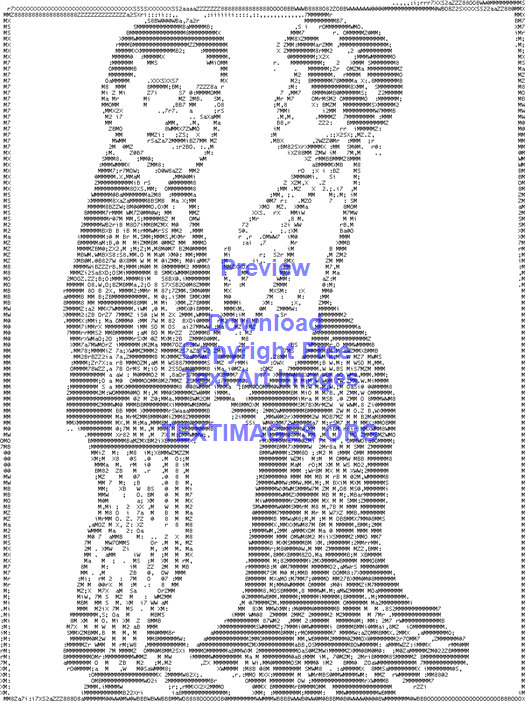The image is a detailed text art creation depicting a man and a woman, generated using a text art website. The man, positioned on the right, faces outward in profile with dark hair, wearing a jacket and pants, creating the illusion of a suit. The woman is on the left, depicted in left-side profile, wearing a long skirt and long sleeve blouse with her hair styled in an updo. She appears to be looking towards the man. The entire scene is meticulously rendered in black and white text characters, forming a clear and recognizable depiction of these two individuals who appear to be around 40 to 45 years old. Overlaid on the central part of the image, blue text reads, "Preview, download, copyright free text art images," followed by the website "textimages.org." This text art is created with letters and numbers, highlighting the intricacy and creativity of the design.